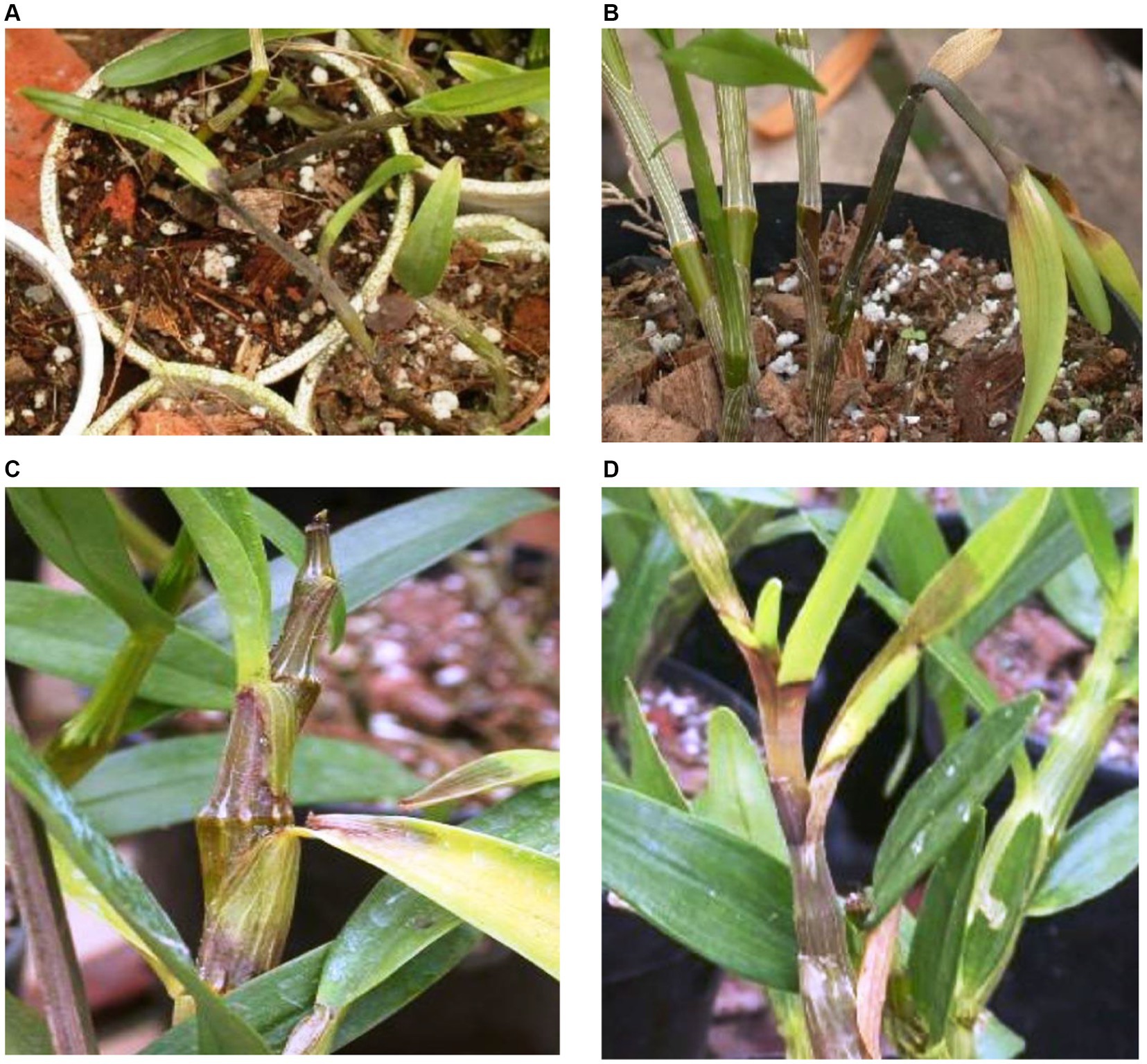This image is divided into four distinct pictures labeled A, B, C, and D with small black text. Each picture captures a different stage in the growth of plants, providing a detailed comparison. 

- In the top-left corner, labeled A, there are five white pots, likely made of styrofoam, each holding soil and a single stem with small, green leaves. Some of these cups are only partially visible.
- The top-right picture, labeled B, features a plant in a black pot with multiple green stems and numerous green leaves, indicating a lush and healthy growth phase.
- The bottom-left image, labeled C, offers a close-up view of a thick plant stem with several leaves, some of which appear to be browning, highlighting a more mature section of the plant.
- Finally, the bottom-right image, labeled D, presents a similar close-up to image C, focusing again on a thick stem with numerous leaves, including new lighter-colored leaves and some browning areas, thus documenting the detailed progression and aging in the plant's lifecycle.